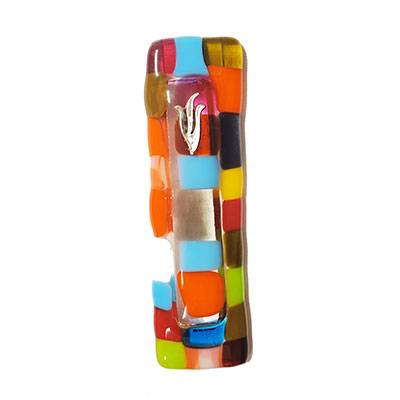The photograph showcases an ornamental piece of fused glass art, characterized by its vibrant array of colors and intricate design. Approximately three to four inches long and around two inches wide, the piece is vertically oriented and prominently features a patchwork-like mosaic of hues. The colors range from clear to opaque with striking shades of pink, blue, amber, orange, black, red, yellow, lime green, and various blues, arranged in a somewhat irregular grid pattern. The grid consists of roughly three colors across and eight colors down, forming a kaleidoscope effect. This decorative item, likely more ornamental than functional, also includes a noteworthy detail: a small sterling silver flame shape affixed at the top center. The glass itself has rounded edges and a glossy surface, enhancing its reflective and eye-catching appeal. Positioned against a solid white background, the piece stands out clearly as the central focus of the composition, inviting viewers to appreciate its artistry and craftsmanship.